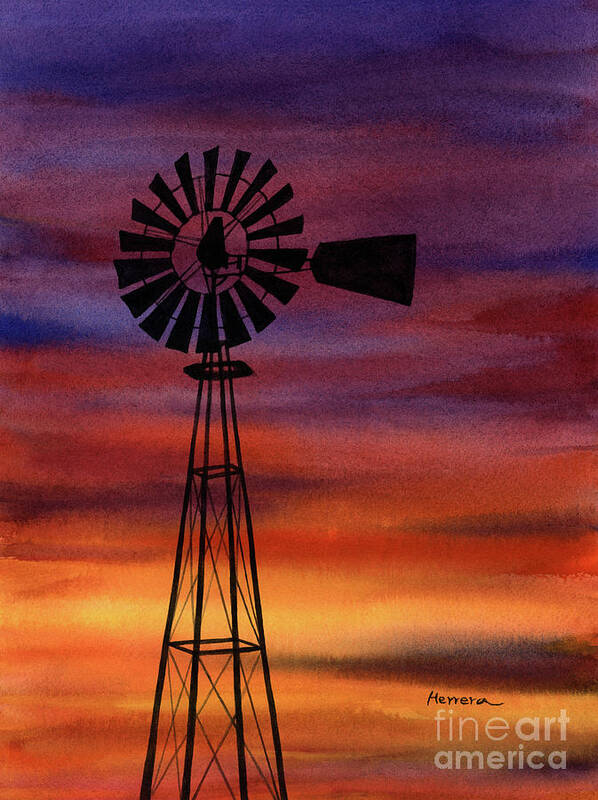This captivating vertical image, photographed by Herrera of Fine Art America, prominently features the striking black silhouette of a tall, thin windmill set against a breathtaking, colorful sky at dusk. The sky transitions through a rich palette starting from deep blues and purples at the top, moving through fiery reds, pinks, and oranges, and tapering off into vibrant yellows and browns towards the bottom. The harmonious blend of these colors vividly captures the essence of a sunset. The windmill, slightly off-center, stands as the main focal point against this vivid backdrop. At the bottom right corner of the image is the artist's signature, "Herrera Fine Art America," with "Herrera" inscribed in black in a distinct font and "Fine Art America" in white.